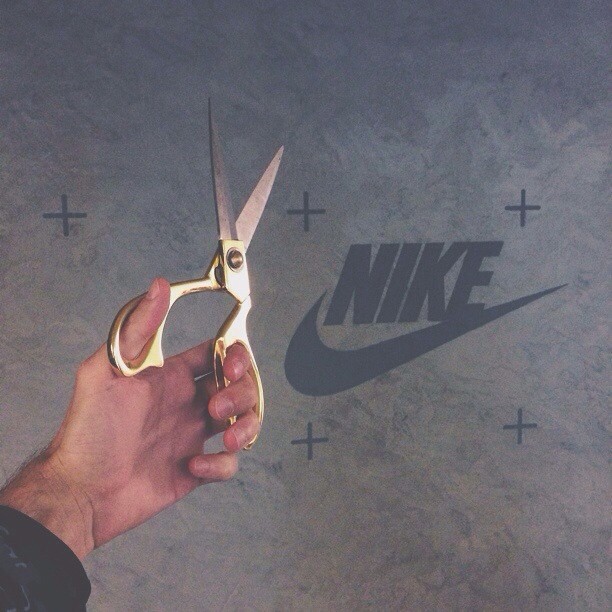A man's left hand, dressed in a dark sleeve, is holding a pair of scissors with golden handles and silver blades, which are currently open. His thumb is through one hole while his index, middle, and ring fingers are through the other. The background is a textured gray, featuring a bold NIKE logo in darker gray, accompanied by the iconic swoosh symbol below it. Five plus signs are visible in the backdrop, with the hand likely obscuring another one. The exact action being performed with the scissors is not clear from the image.